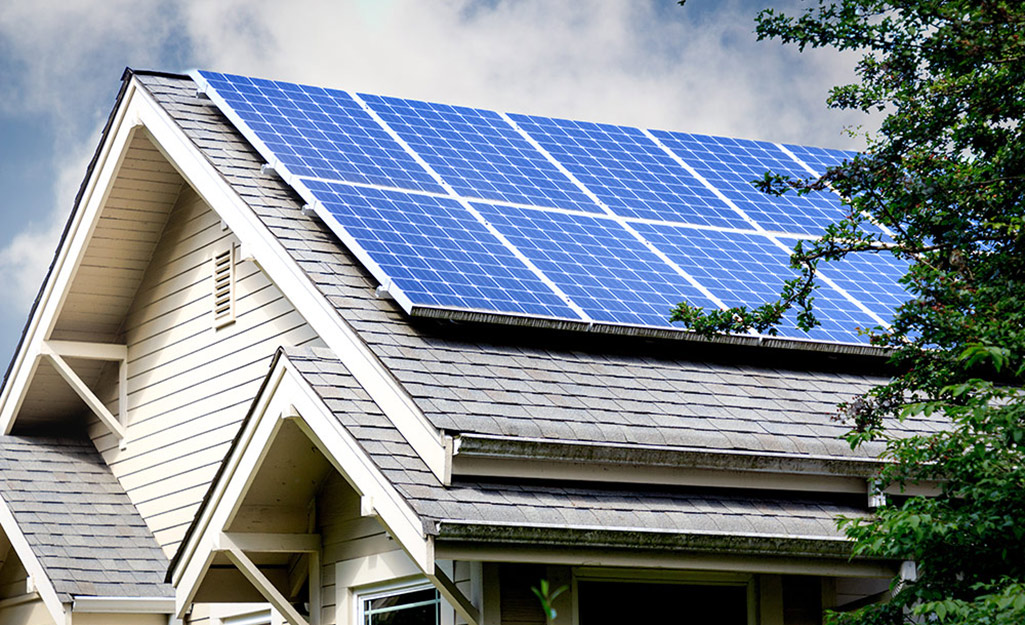The digital photograph captures the roof of a house prominently adorned with eight blue solar panels, each outlined in white metal. The A-shaped roof, composed of gray shingles, features a secondary smaller roof beneath which the top of the front door is visible. The solar panels, designed with a grid of squarish sections, almost completely cover the roof, highlighting the emphasis on energy conservation. Surrounding the house, vibrant green trees suggest that the season is summertime. In the background, a dark blue sky with wispy clouds adds depth to the scene. The house itself is off-white, almost tan, with notable white hardy boards on the front. The meticulous detailing of the solar panels and the surrounding environment underscores the artist’s intention to promote the integration of renewable energy.